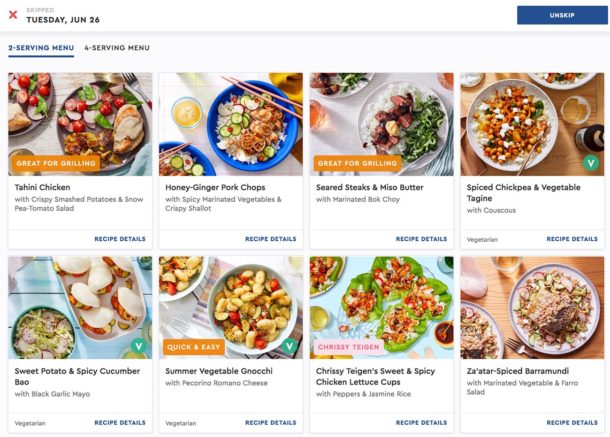The website showcases a variety of food dishes organized for a meal menu selection. In the upper left corner, a red X icon is positioned next to the word "Skipped," with "Tuesday, June 26th" displayed prominently in bold font. In the upper right corner, there is a blue button labeled "Unskip" in white font.

Below this section are options for "2-Serving Menu" and "4-Serving Menu," with the "2-Serving Menu" currently selected. The page features eight meal options, arranged in two rows of four, each accompanied by an appetizing photograph above its description.

1. **Tahini Chicken** – Served with crispy smashed potatoes and a snow pea tomato salad.
2. **Honey Ginger Pork Chops** – Paired with spicy marinated vegetables and crispy shallot.
3. **Seared Steak and Miso Butter** – Accompanied by marinated bok choy.
4. **Spiced Chickpea and Vegetable Tagine** – Served with couscous.
5. **Sweet Potato and Spicy Cucumber Bao** – Featuring black garlic mayo.
6. **Summer Vegetable Gnocchi** – Topped with Percorino Romano cheese.
7. **Chrissy Teigen's Sweet and Spicy Chicken Lettuce Cups**
8. **Za'atar Spiced Barramundi** – Served with marinated vegetables and farro salad.

Each dish option includes a link for more details, indicated by blue text labeled "Recipe Details."